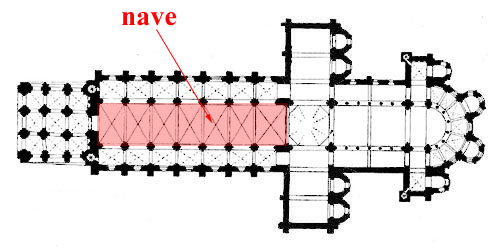The image is a detailed floor plan, likely for a church, featuring a blend of colors, primarily reds, pinkish-red, black, and white. The design looks computer-generated, evident from its pixelated, perfectly straight lines. Notably, the plan highlights a long central corridor, which extends from the left and culminates in an arched, semi-circular end on the right. Midway along this main corridor, two hallways branch off to the top and bottom, resembling wings. A pinkish-red rectangle is prominently marked on the left side of the corridor. A bold, red arrow points to this area, and in lowercase Times New Roman font, it reads "nave." This term, associated with church architecture, indicates the central part of the church where the congregation typically sits. The floor plan, detailing both the layout and key features, suggests a meticulously designed church interior.